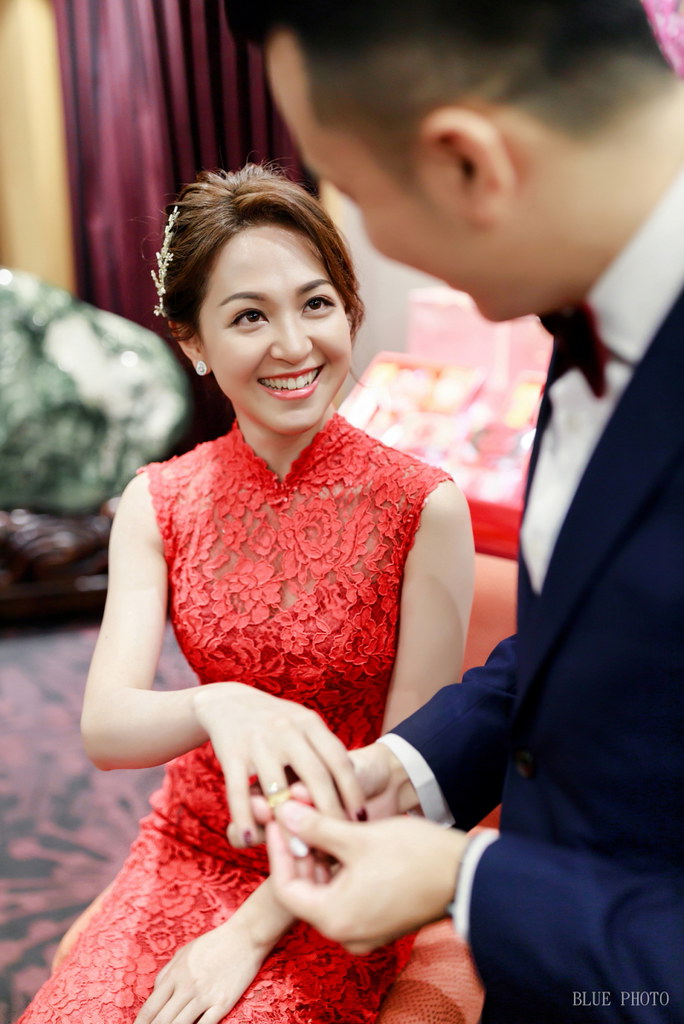In this indoor photograph, captured in portrait mode, we see an intimate moment between a man and a woman, presumably a couple, both of Chinese ethnicity. The woman, seated at the center of the image, is wearing a bright red lace sleeveless dress with a high collar, accentuated by silver barrettes in her long, highlighted brown hair, and matching silver earrings. She is looking up at the man with a radiant smile, showcasing her upper teeth adorned with pink lipstick. The man stands slightly to the right, bending towards her as he carefully places a ring on her finger. He is dressed in a blue dress jacket over a white shirt and teal bow tie, though his face is slightly blurred. His black hair is neatly cut short. The background, intentionally blurred to emphasize the couple, hints at a formal event with red curtains, a green settee, a table, and a gray and pink patterned carpet. The photograph is watermarked with "blue photo" in the bottom right corner.